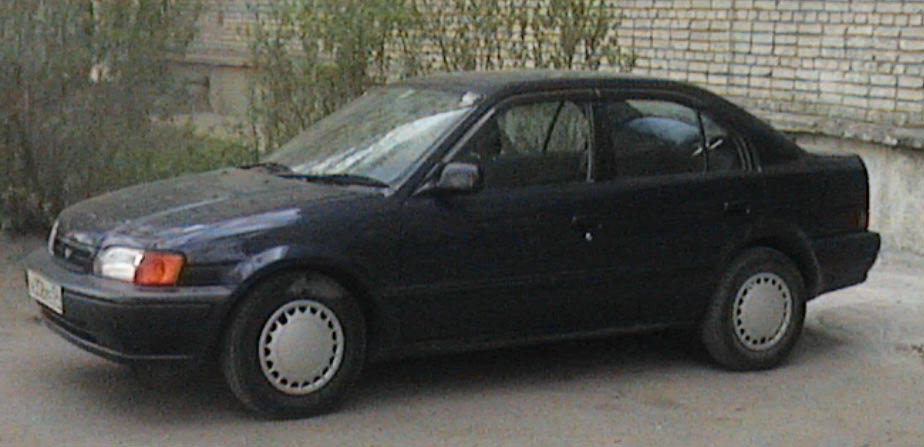This is a detailed side view of an older model small sedan, likely from the late 80s or 90s, parked on a concrete driveway. The car is dark navy blue or possibly black, with gray hubcaps and a black bumper. The vehicle appears somewhat dusty, indicating it hasn't been driven recently. Its interior is a dark color, perhaps black or dark blue, though it’s difficult to see clearly due to the graininess of the photo. The car's windshield also appears dusty. The front end of the car is directed towards the right, with its rear facing left. The front license plate is visible but unreadable, and the headlights seem to be on, appearing slightly bright. 

In the background, there’s a solid brick wall in a dirty beige-gray hue with hints of light pink streaks, possibly the exterior of a building. To the right side of the car, there are small trees or tall plants with green leaves. The scene is rather plain, without any text or notable features, concentrating on the gritty, compact, and slightly worn look of the vehicle against a simple backdrop.